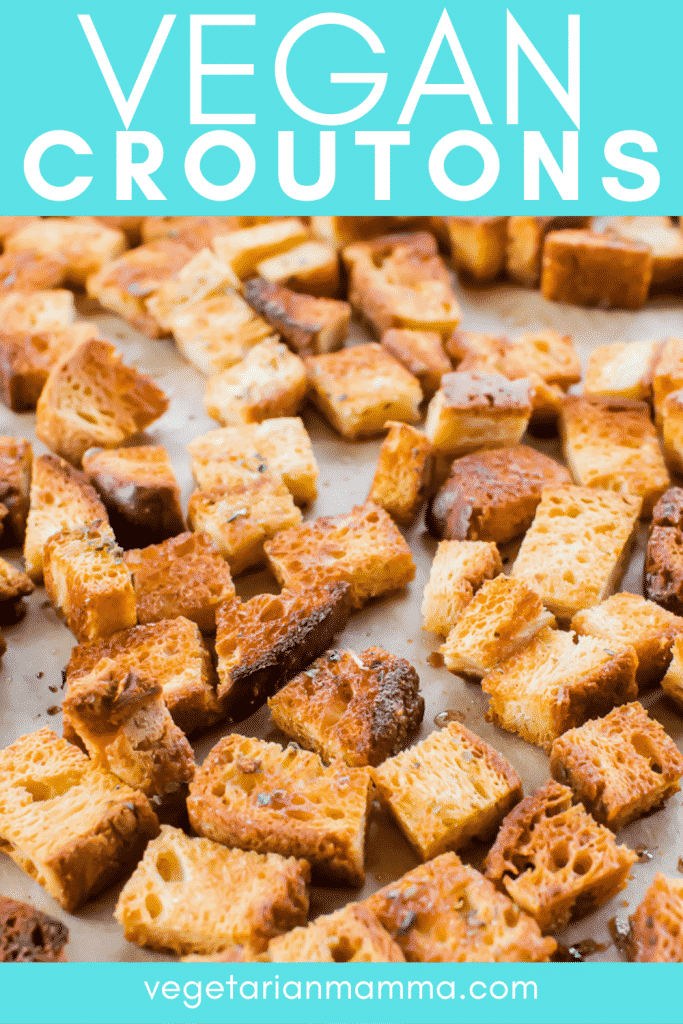The image prominently features a close-up of croutons, showcasing their toasted and lightly browned textures. The croutons, some of which are almost burnt and others a pale golden color, are arranged on what seems to be a metal baking sheet. Small droplets of oil and hints of herbs are visible, adding detail to their appearance. The background highlights two teal-colored stripes: the top stripe displays "VEGAN CROUTONS" in large, white all-caps font, while the bottom stripe, in a smaller white font, reads "vegetarianmama.com". This detailed layout suggests a vegan crouton recipe or advertisement from the website vegetarianmama.com.